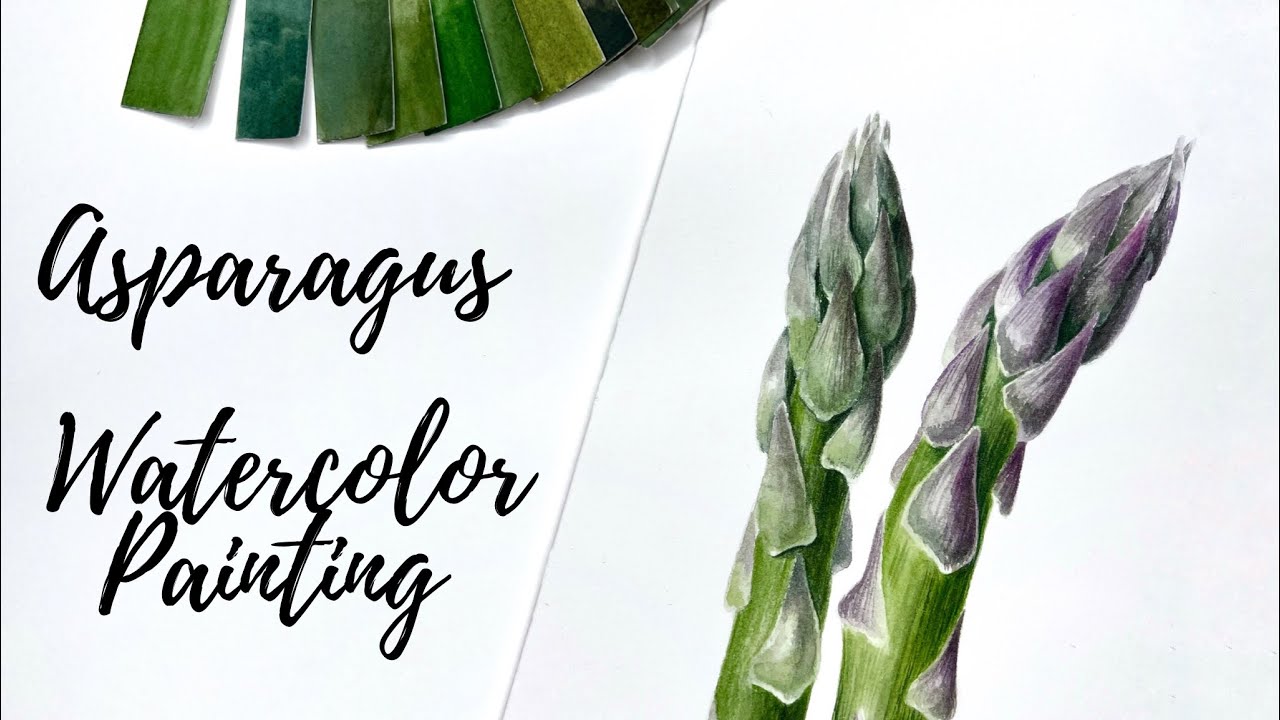The image features a split diagonal composition, predominantly against a white background. On the top-left corner, various green paint swatches resemble stick shapes, hinting at different shades. Below this, elegant black cursive script reads "Asparagus Watercolor Painting," indicating a tutorial or advertisement. The right side showcases a detailed watercolor depiction of two asparagus spears, arranged vertically. The spears display a realistic blend of light greens and purples, particularly at the tips, capturing the delicate transition of colors. The overall aesthetic suggests the image could be an introductory visual for a painting tutorial website or possibly a book cover dedicated to watercolor techniques.